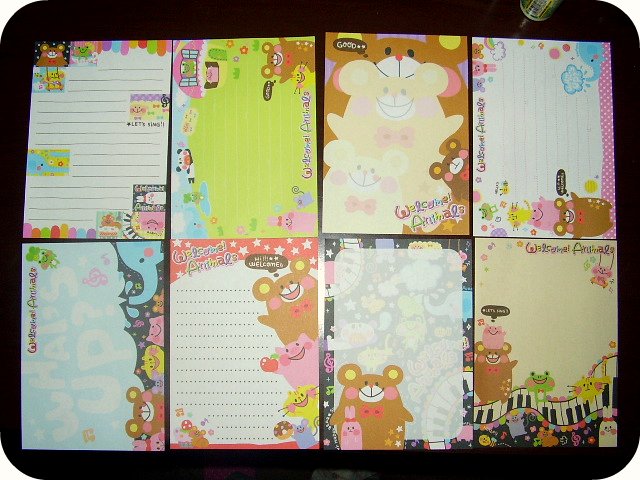This photograph features eight distinct notepads arranged in a grid of four on the top row and four on the bottom row, set against a dark brown or black background. Each notepad is adorned with whimsical cartoon illustrations and lined pages, reminiscent of children's notebook pages. The notepads vary in orientation, with some arranged lengthwise and others horizontally. Prominent among the illustrations are cartoon-style teddy bears, presented in muted blues, pinks, oranges, and yellows, along with other animals such as blue elephants, green frogs, yellow birds, and pink rabbits. Several notepads feature the repeated phrase "Welcome Animals" in a playful script. The top-left notepad is mostly white with a teddy bear image in the top-left corner. A neighboring notepad has a light green background and is positioned on its side. Another notepad presents a pink and white polka dot strip. The collection includes a variety of designs, displaying a mix of light blue, white, tan, and black tones, with one particular notepad featuring a piano motif in the bottom right-hand corner. The overall visual effect is a charming and juvenile aesthetic, perfect for kids or anyone who enjoys cute and playful stationery.